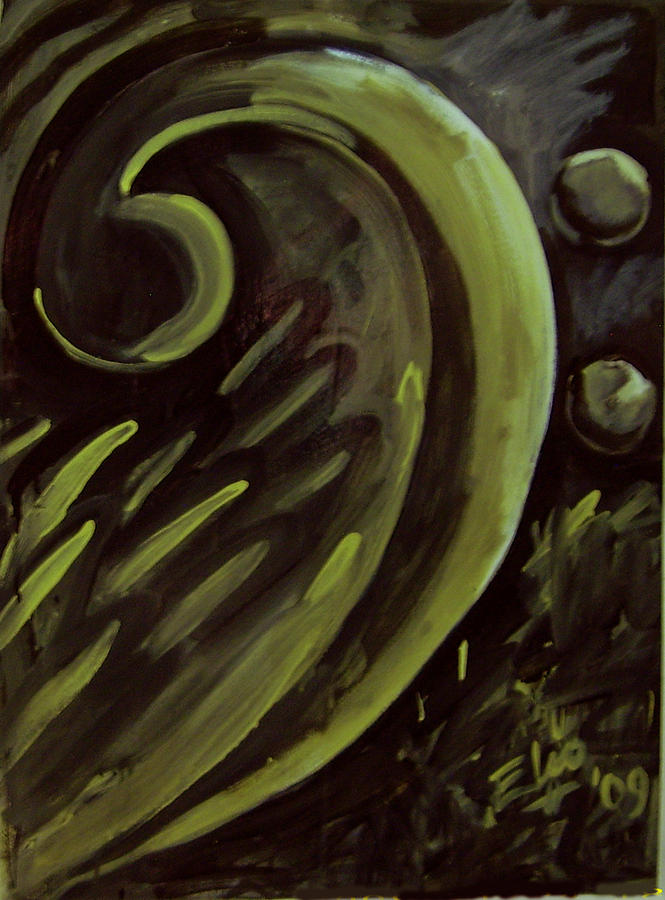This detailed photograph captures an abstract painting predominantly in shades of green and black, signed "E. Liu 09" in the bottom right corner in a lighter green or grayish neon paint, indicating it was created in 2009. The painting features a prominent green swirl starting from the bottom left corner, rising upwards and curling into a hook shape at the top left. Within this swirl, brush strokes resemble grass, suggesting a botanical theme. To the right of this main element, multiple green, pod-like circular shapes float around, contributing to the abstract composition. A messier green area at the bottom right appears as additional vegetation or grass. The overall dark background accentuates the green elements, creating a vivid contrast. Hints of brownish-red, gray, and possibly yellow also contribute to this richly textured and imaginative artwork.